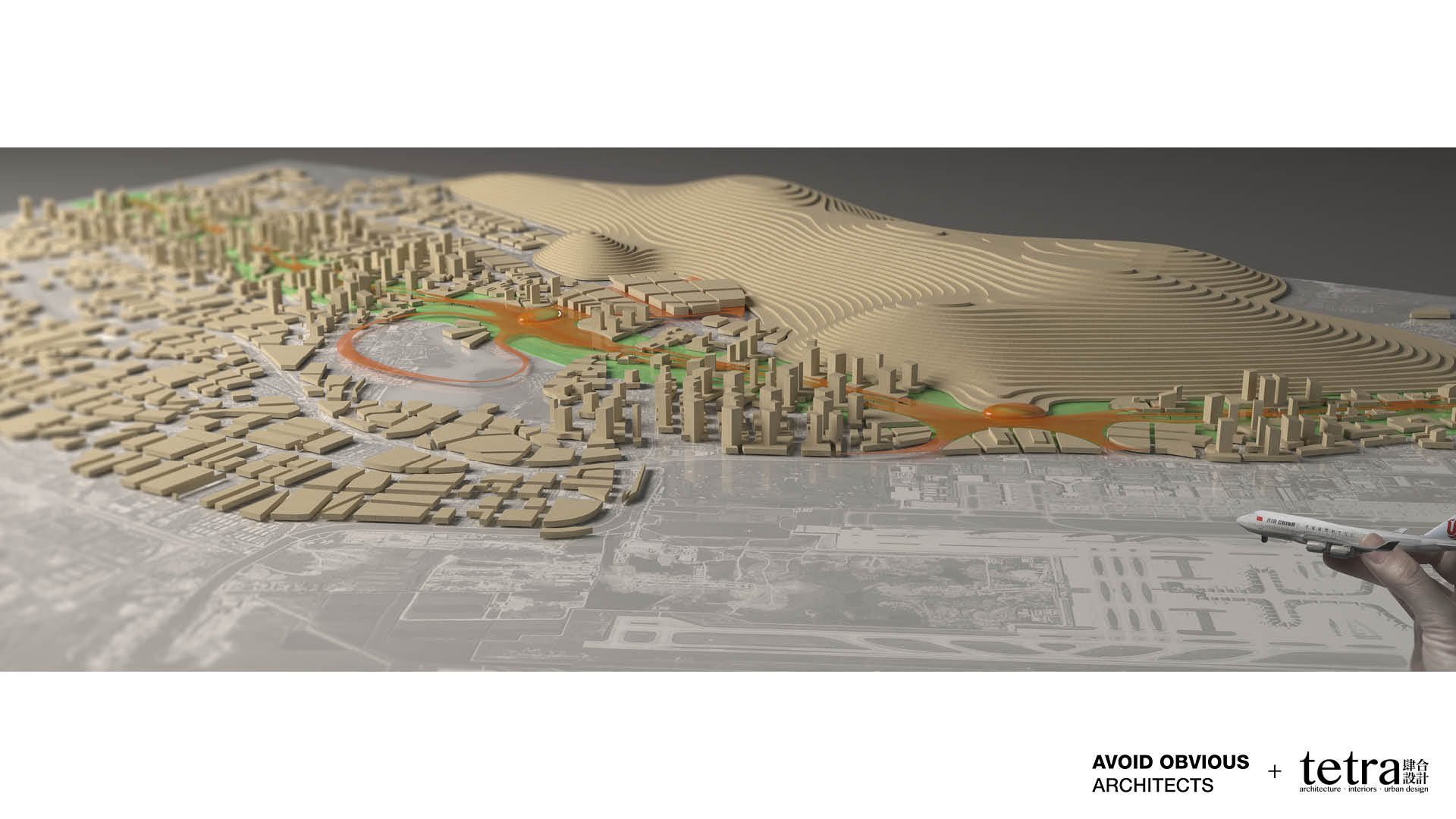The image showcases an intricate architectural model from an aerial viewpoint, depicting a cityscape seamlessly integrated into a desert environment. Dominating the top half of the image are detailed blueprints of the city, which include a mix of beige rectangular buildings and verdant areas represented by light green hues, suggesting urban planning with landscaped spaces. As the eye moves up from the bottom left to the upper regions of the image, the buildings increase in density and height, indicating a varied skyline. On the right side, a distinctive orange ground snakes through, presumably depicting pathways or roads, and is juxtaposed against areas of lime green, possibly symbolizing vegetation or parks. The backdrop features a dark gray horizon, likely signifying the sky, which contrasts with the light gray and beige tones of the foreground. In the bottom right corner, a model airplane is held aloft, adding a dynamic element as if in flight over the model, embodying futuristic aspirations. The text overlay reads "Avoid Obvious Architects plus Terra," enhancing the conceptual blend of urban design within a natural landscape. The overall setting exudes a visionary architectural design, combining elements of city planning with the natural desert terrain, rendered in a palette of orange, lime green, beige, white, red, and various shades of gray.